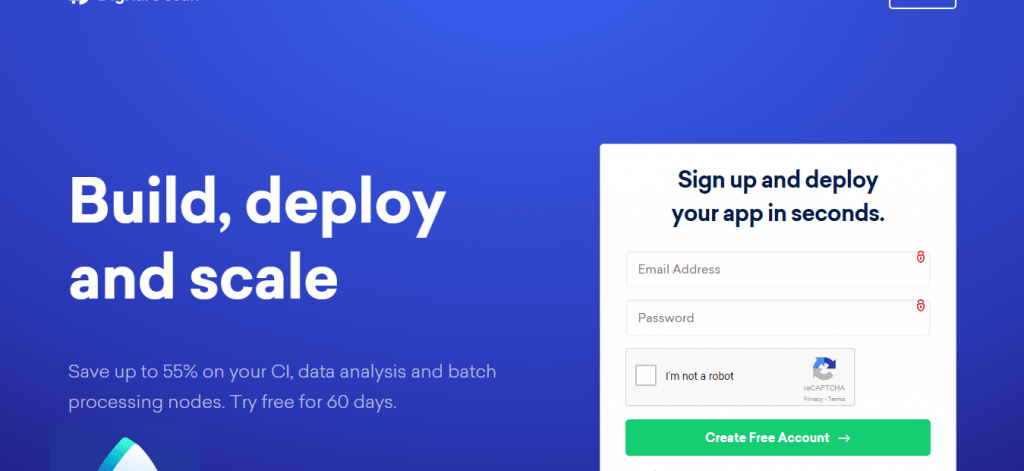This partial screenshot features a blue background with prominent text and a sign-up dialog. On the left side, in large white font, the text reads "Build, Deploy, and Scale". Below this, there's a smaller font that promotes, "Save up to 55% on your CI, data analysis, and batch processing nodes," followed by an invitation to "Try free for 60 days." A partially visible logo is located beneath this text.

On the right side of the screenshot, there's a white dialog box with black text that instructs, "Sign up and deploy your app in seconds." The dialog includes an input field for an email address, another for a password, and a reCAPTCHA feature labeled "I'm not a robot" with a corresponding checkbox. At the bottom of the dialog is a large green button featuring a white arrow pointing to the right and the text "Create Free Account" in white font.

Additionally, at the very top right of the blue background, there is a partially visible outline of what appears to be a button. On the top left, a few small white elements hang down, adding to the overall details of the image.